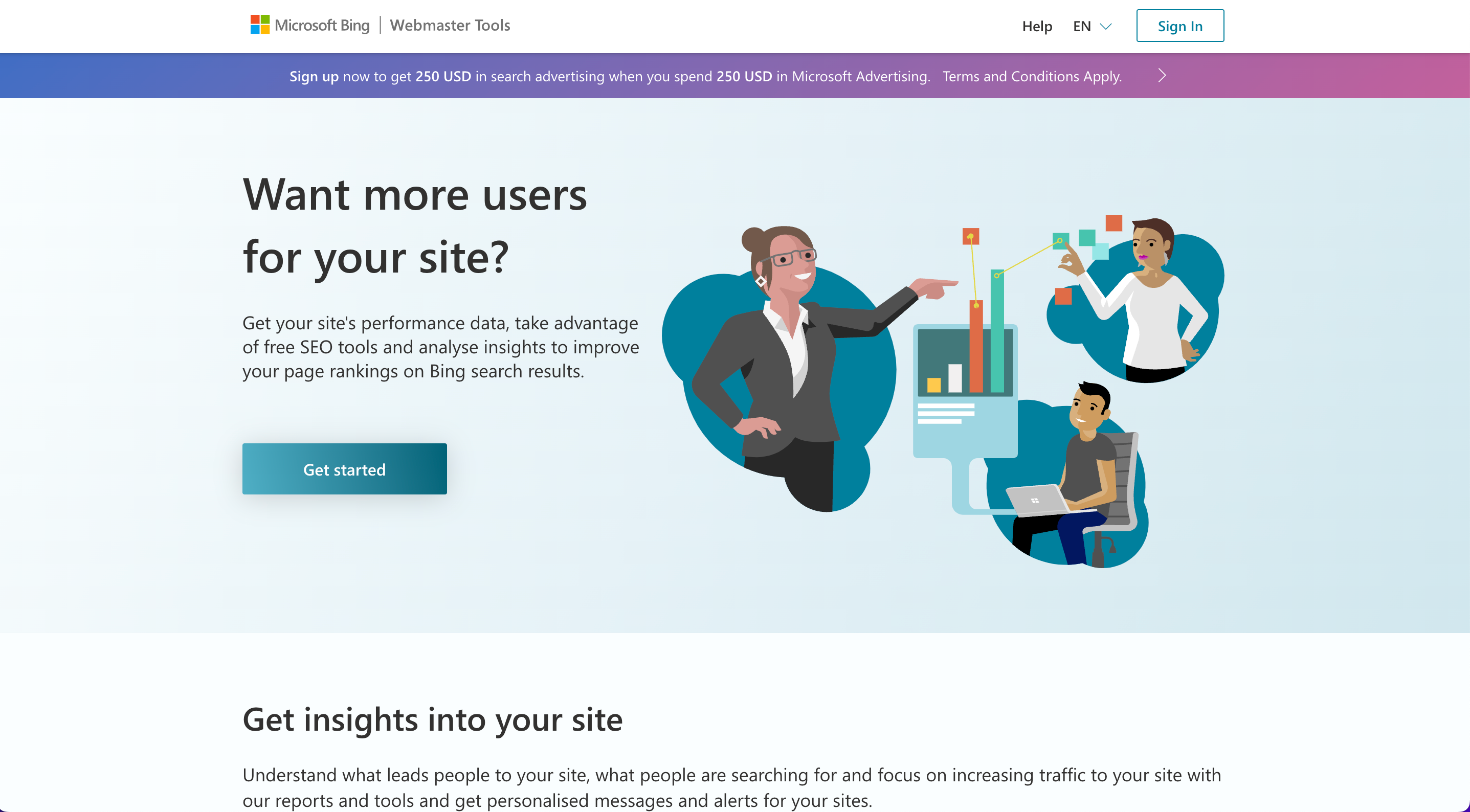**Detailed Caption for Homepage Screenshot of Microsoft Bing:**

This is a screenshot capturing the homepage of Microsoft Bing. Dominating the top left corner is the Microsoft logo, followed by the text "Microsoft Bing" in small black letters. A tiny vertical line separates "Microsoft Bing" from the adjacent "Webmaster Tools." Moving rightwards, there are several navigational options: a help link, a language drop-down menu defaulted to English, and a blue rectangular sign-in button emblazoned with "Sign in" in blue text.

Directly beneath this menu bar is a prominent gradient purple banner urging visitors to "Sign up now to get $250 USD in search advertising when you spend $250 USD on Microsoft advertising." This offer is accompanied by a disclaimer—"Terms and conditions apply"—and ends with a rightward-pointing arrow for emphasis.

Central to the webpage layout is a vast gradient blue-to-light-blue box. Positioned to the left within this box is the headline, "Want more users for your site?" in large, bold black letters. Below this, there's an invitation to "Get your site's performance data, take advantage of free SEO tools, and analyze insights to improve your page rankings on Bing search results." A blue "Get Started" button is prominently placed below this call to action.

To the right of this central message, there is a visual element: a click bar featuring an image of people collaboratively working, depicting a professional work environment.